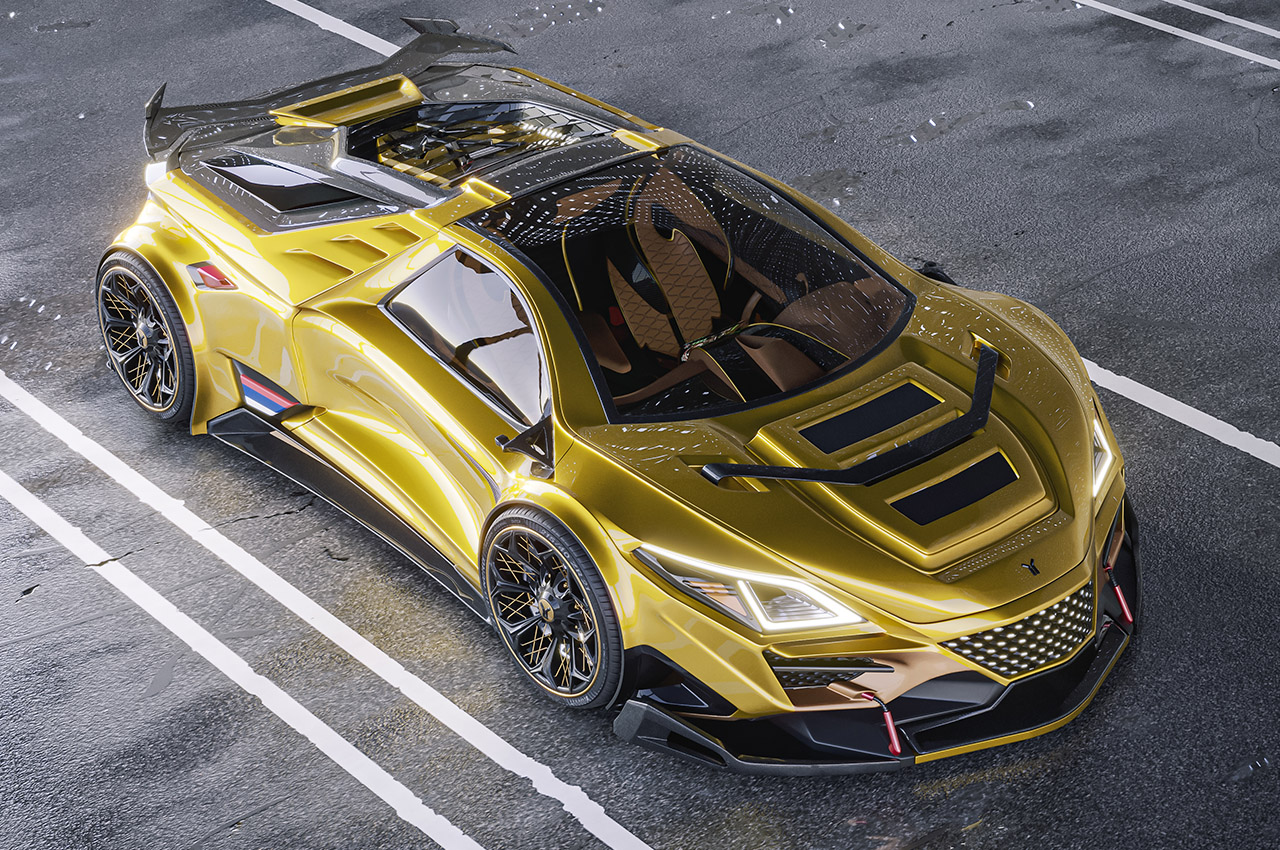This image features a striking golden yellow sports car, parked neatly within a designated parking spot on an asphalt surface. The parking area is clearly defined by crisp white lines. The car, boasting an undeniable air of luxury and speed, features only two seats—suggesting a sleek, performance-oriented design. The wheels are black with intricate golden yellow detailing that gives them a complex, web-like appearance. The interior appears to be a sophisticated tan or light brown with subtle black accents, adding to the car’s elegant yet sporty aesthetic. The vehicle's exterior is highly polished, reflecting a glossy shine, and includes black accents that complement its vibrant color. Although the exact brand of the car is indiscernible, its overall design, including what seems to be a hatchback, emphasizes its high-performance capabilities and exclusivity. The image itself is so finely detailed that it almost appears computer-generated, adding an extra layer of intrigue to this captivating depiction of automotive excellence.